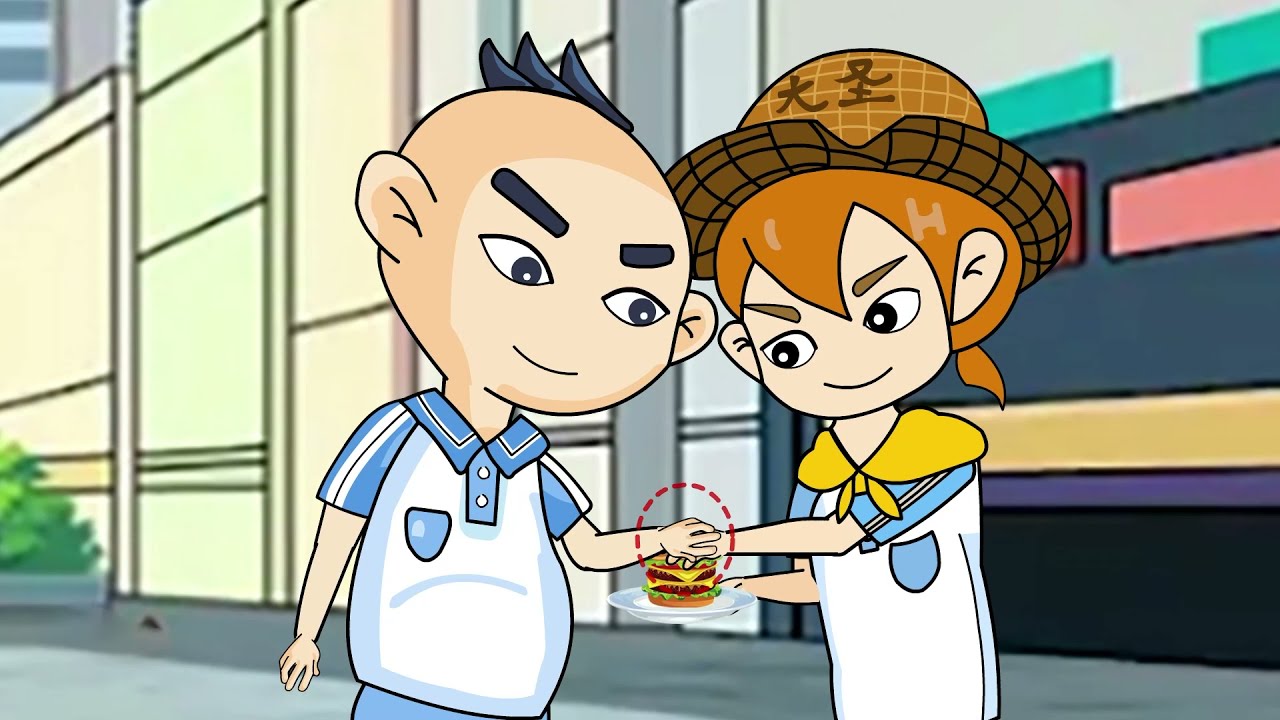This is a cartoon image featuring two characters standing in what appears to be the middle of a city street. Both are wearing identical white polo shirts that have blue trims around the collar and sleeves, as well as blue pockets. The character on the left is mostly bald, sporting some black hair sticking up in the center of his head like a mohawk, and has black eyebrows with a little grin on his face. The character on the right, wearing a brown straw hat with Chinese writing, has shoulder-length red hair tied back in a ponytail, thin brown eyebrows, and is accessorized with a mustard-yellow cape or scarf around her neck. Both characters have their hands touching a large double-meated cheeseburger that the girl is holding on a plate. Their poses suggest they are either attempting to share or simultaneously grab the cheeseburger. The background includes some buildings and a tree situated to the left.